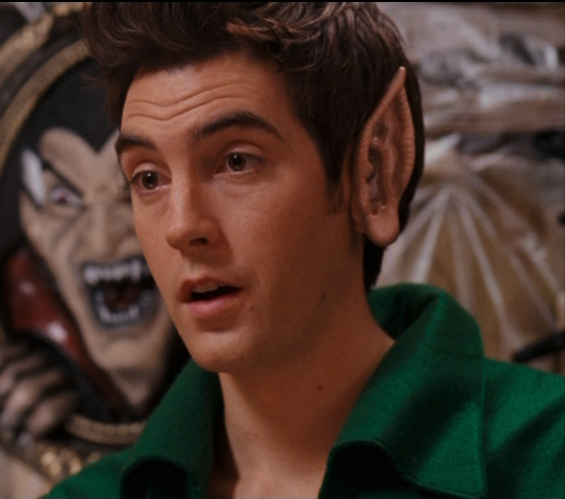In this detailed photograph, a man who appears to be in his twenties or early thirties is dressed in an elaborate green costume, complete with a ruffled shirt featuring a large, pointy collar. His pale complexion contrasts with his styled brown hair, which is fashioned to have his bangs pointed upwards. He wears impressively large, pointed prosthetic ears made from plastic or silicone, reminiscent of those of an elf or Vulcan. The image captures him from the shoulders up, highlighting his expressionless face. In the background, slightly out of focus, is a mural or decorative artwork depicting a frightening figure with a widow's peak hairstyle and fangs, possibly hinting at a vampire or a monster. This setting, combined with his costume, suggests that the scene might be from a movie or television show, or alternatively, could have been taken in a themed environment such as a Halloween shop.